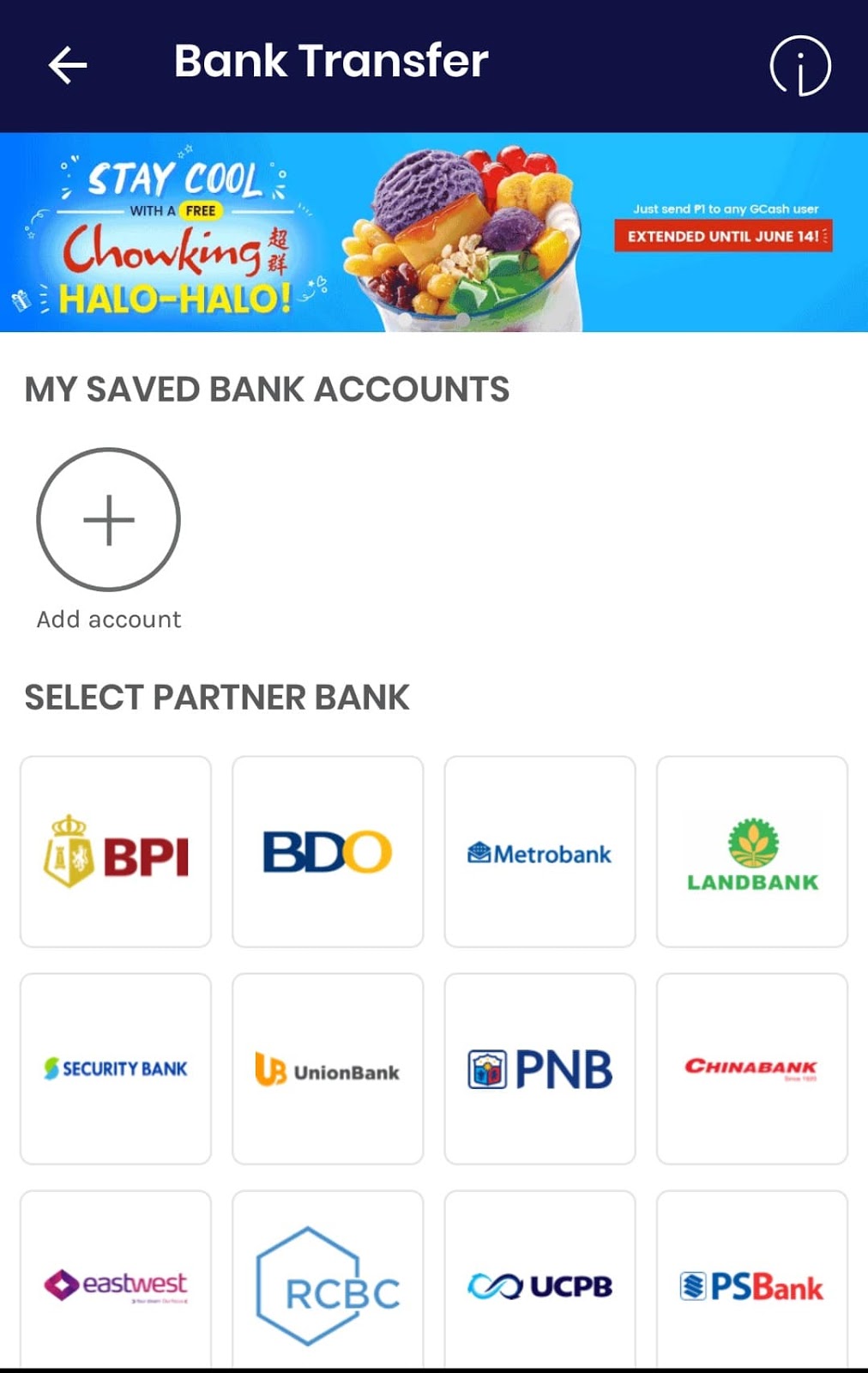**Image Description:**

The image is a detailed screenshot of a bank transfer interface with a promotional section for a dessert.

**Top Section:**
- **Background:** Dark blue
- **Text:** "Bank Transfer" written in white at the top-center
- **Icons:** 
  - A back button on the top left, drawn in white
  - An information icon on the top right, also in white

**Promotional Banner:**
- **Background:** Blue
- **Text:**
  - "Stay cool with the free" written in white
  - "choking" written in red
  - "hallo hallo" written in yellow
- **Image:** On the right side, a cup filled with a colorful dessert consisting of purple ice cream, red creams, and green cubes
- **Additional Text:** "Just send P1 to any Gcash user"
- **Button:** Red button with white text that says "Extended until June 14th"

**Main Page:**
- **Background:** White
- **Text on the left side:**
  - "My Saved Bank Account" written in black
  - Below it, a circle with a plus sign labeled "Add Account"
  - Further down, "Select a Bank" with a grid of bank options
- **Bank Options (12 total, labeled):**
  - Top row (left to right): BPI, BDO, Metro Bank, Land Bank
  - Middle row: Security Bank, Union Bank, PNB, China Bank
  - Bottom row: EastWest, RCBC, UCPB, PS Bank (bottom right)

This comprehensive structure of the content effectively illustrates the user interface and promotional aspects of the image.